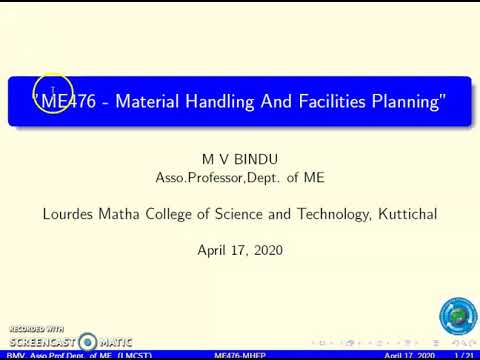The image is a wide rectangular screenshot of a PowerPoint presentation, featuring a blend of white, blue, and beige colors with black, white, and yellow text. At the top, there is a prominent blue banner with curved edges and a shadow, containing the white text "ME 476 - Material Handling and Facilities Planning." A yellow circle highlights the "ME 476" part. Below this banner, in black text, it reads, "M.V. Bindu, Associate Professor, Department of ME, Lourdes Matha College of Science and Technology, Kutichal." The date "April 17, 2020" appears twice in the image, once in the body of the slide and once in the bottom right corner, accompanied by additional, small, hard-to-read text. At the bottom of the image, there's a thin blue strip, and the word "Screencast-O-Matic" is visible, likely indicating the screenshot's origin. Additionally, a small earth symbol is present at the bottom right. The background of the main slide is beige with blue and green accents, providing a clean and professional layout typical of academic presentations.